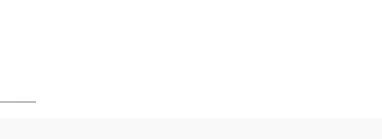In this minimalist image, the background is a pristine white. The only items present are a short, thin gray line situated at the bottom edge of the frame, though it could also be interpreted as the top edge depending on perspective. Above this line lies a light-shaded gray rectangle that spans the entire width of the image from left to right. This rectangle appears to be a placeholder for information.